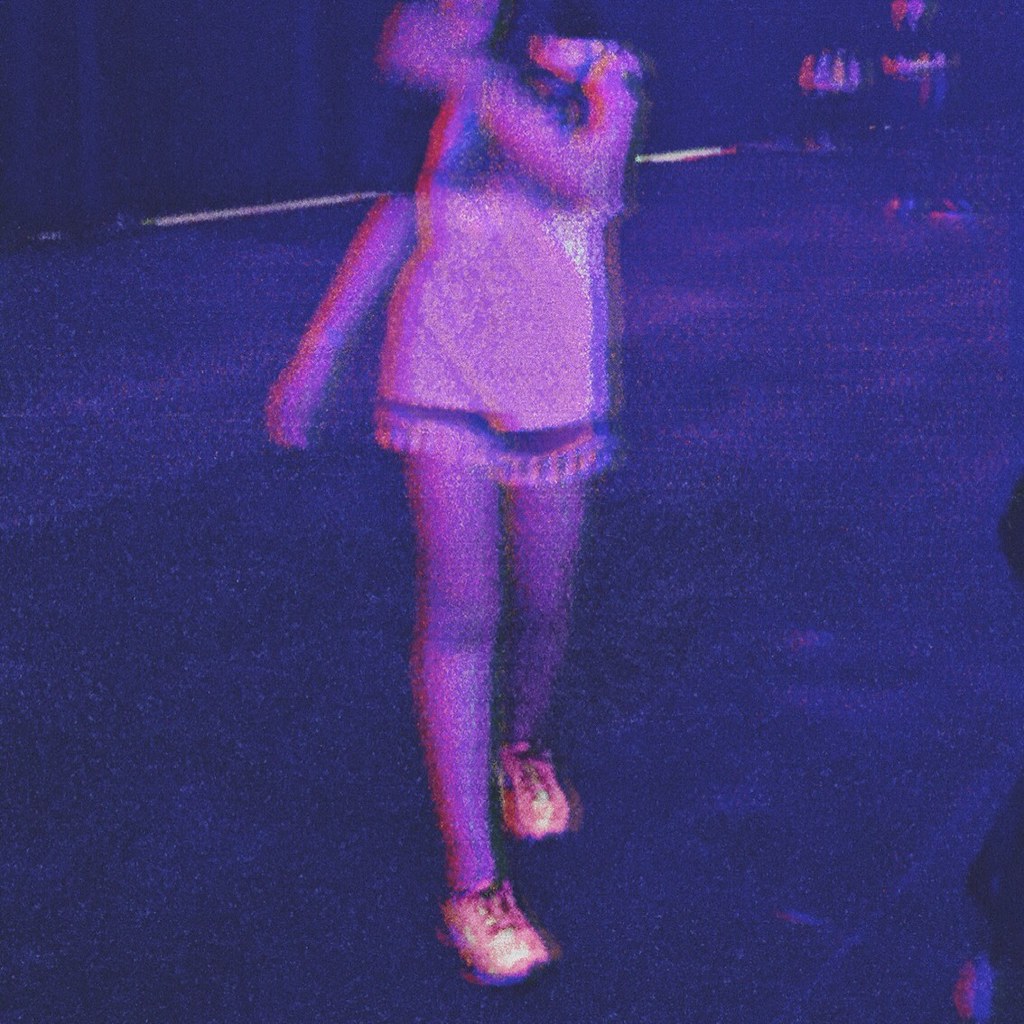The image depicts an out-of-focus, nostalgic scene reminiscent of an old school photograph displayed on a CRT TV. At its center is a woman wearing a white, short dress adorned with delicate designs that dangle down her legs. Her bare arms and legs contribute to an ethereal quality, and one arm crosses her body, holding an indistinguishable object to her face in a manner that creates an illusion of detachment. She stands on a floor that appears to be made of stone or concrete, while her bright white shoes starkly contrast with the muted tones surrounding her. The back wall has a peculiar detail with a patch of white emerging from its base, adding to the overall dreamlike and somewhat puzzling atmosphere of the image.